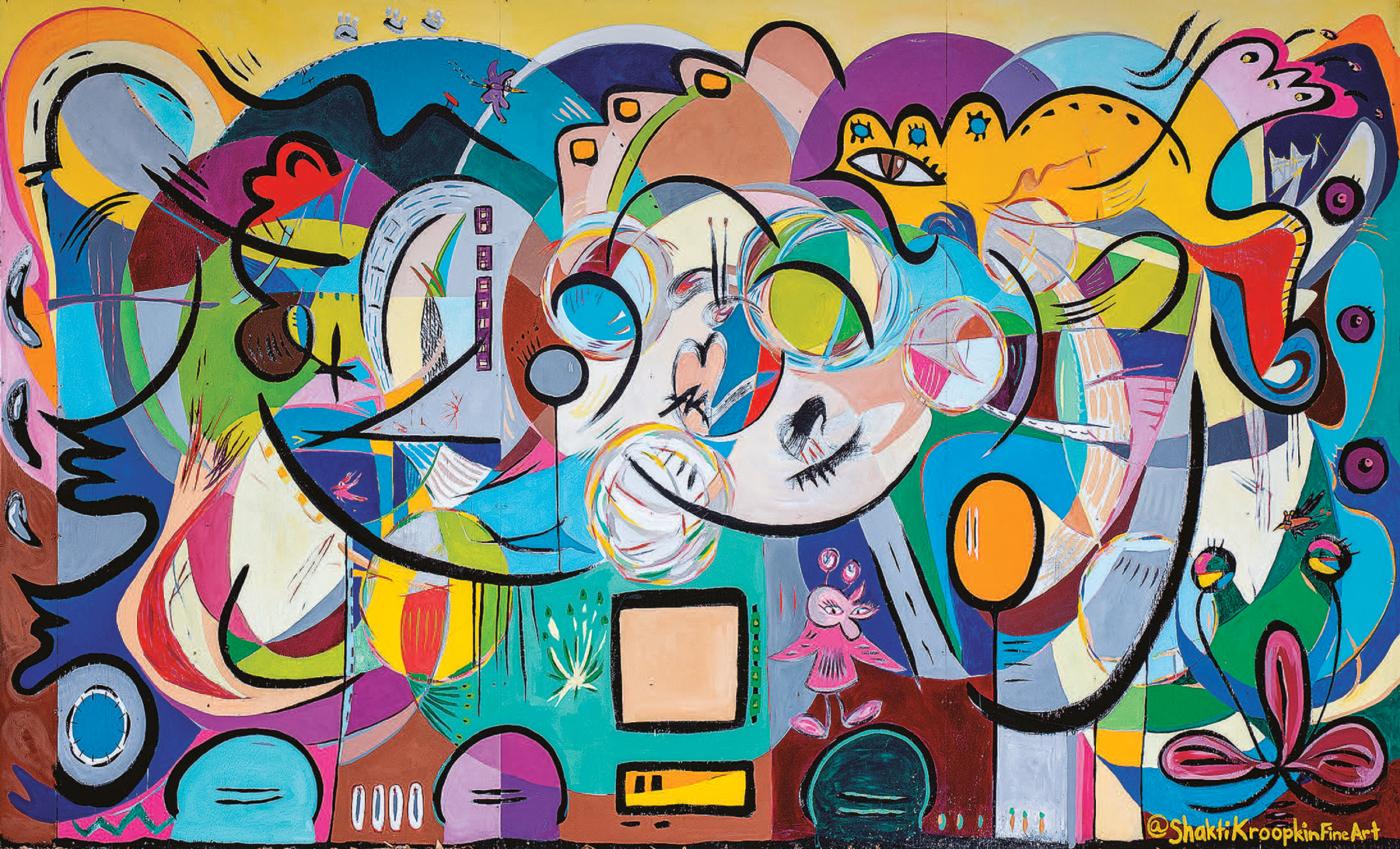This vibrant and chaotic abstract art piece, seemingly a modern homage to Picasso with echoes of the tumultuous energy of "Guernica," is attributed to Shakhty Krupin Fine Art. The overall composition is dominated by a bright and diverse color palette including pinks, purples, blues, greens, yellows, reds, and browns, accented by bold, dark, graphic lines that organically meld and create shapes throughout the artwork.

The image features an interplay of overlapping and overlaying shapes, providing a complex and dynamic viewing experience where different elements and forms become apparent depending on the angle one views it from. Notably, there are intermittent figures and motifs such as eyes, a peculiar pink bird-like creature with antennae positioned at the bottom, and what appears to be purple, flower-like plants on the right side. These elements give the piece a sense of movement centralized in the heart of the composition, drawing the viewer's eye into a vivid, detailed world where every glance may reveal something new and unexpected amidst the chaos.